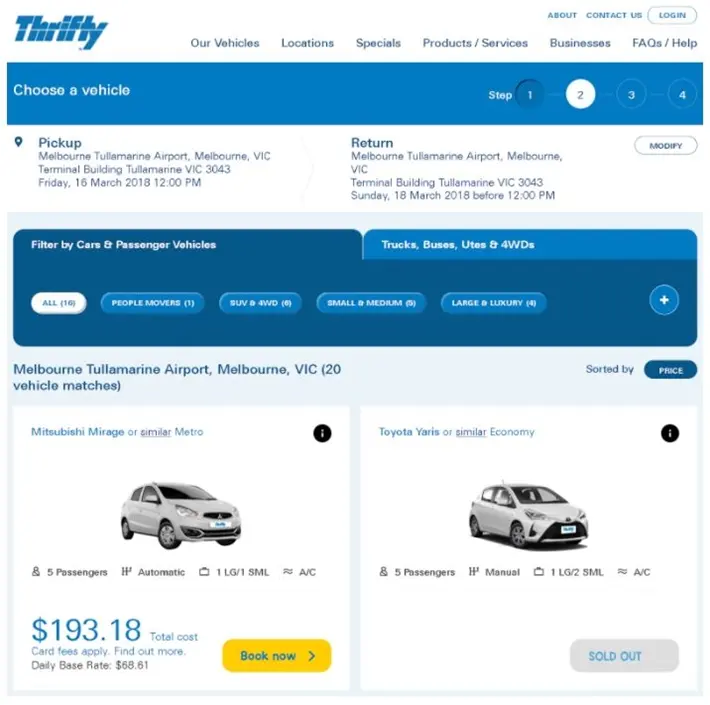The image captures a screen grab from the Thrifty website displayed on a vertically oriented, slightly rectangular frame. At the very top left, the iconic Thrifty logo is prominently featured in blue on a white upper banner. Positioned at the upper right corner of this banner are navigation links labeled "About," "Contact Us," and "Login."

Beneath this, an additional navigation menu spans horizontally, showcasing tabs labeled "Our Vehicles," "Locations," "Specials," "Product Services," "Businesses," "Faq," and "Help." Immediately below this, a blue horizontal banner with white text reads "Choose a Vehicle." To the right of this banner, a sequence of steps labeled "Steps 1, 2, 3, and 4" is displayed, with Step 1 appearing indented to symbolize its completion and Step 2 highlighted in yellow to indicate the current step.

Just below, pickup locations "Melbourne, Tullamarine Airport, Melbourne BIC" are listed, accompanied by “Return Information” on the right side. Two tabs are visible under this section: "Filter by Cars and Passenger Vehicles" and "Trucks, Buses, UTs, and Four-Wheel Drives." The "Filter by Cars and Passenger Vehicles" tab is currently active, with two side-by-side images of vehicles displayed underneath.

On the left is a Mitsubishi Mirage, priced with a total cost of $193.18, accompanied by a "Book Now" button. To the right is a Toyota Yaris, where the selection button at the bottom indicates that it is "Sold Out."